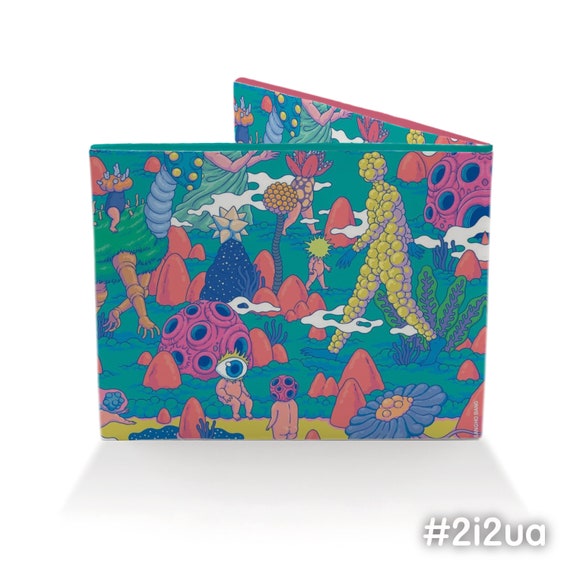The image depicts a vividly detailed paper booklet, designed with a vibrant, abstract depiction of an underwater alien marine world. The booklet, which appears to have two covers, front and back, features whimsical and surreal futuristic imagery reminiscent of a fantastical, otherworldly scene from a "Rick and Morty" episode. At the bottom of the cover, there is text that reads '#2i2ua' or '212 UA'. 

In this psychedelic underwater world, there are bizarre figures such as babies with enormous eyeball heads, toddlers with coral-like heads, and another child-like figure sporting a star-shaped head. Among these strange beings, there's a character entirely composed of a yellow sphere from head to toe, with the exception of its leaf-like green claw hands and feet. The scene is awash with bright, multicolored components—yellows, reds, oranges, pinks, blues, greens, blacks, and whites—creating a chaotic yet captivating visual experience. Additionally, there are various multicolored organisms, including an array of plants and a large, colorful worm featuring shades of yellow, green, purple, tan, and blue, contributing to the overall surreal and fantastical quality of the imagery.